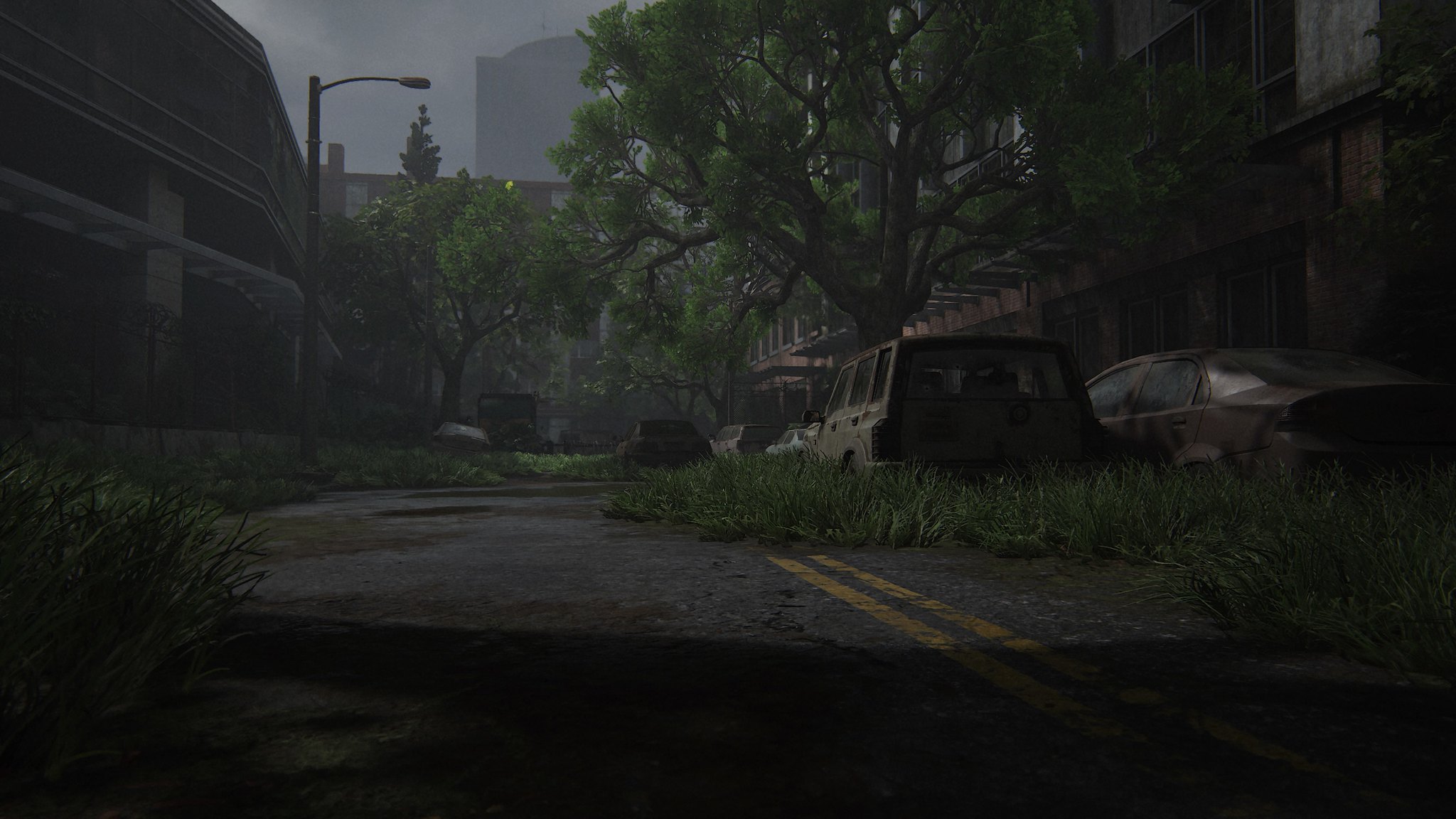The image depicts a desolate urban area reminiscent of an apocalyptic setting, often seen in high-end, modern video games like The Last of Us. The overall tone is gritty and gray, imbuing the scene with a sense of despair. The street, once paved with black asphalt marked by a double yellow line, is now largely overtaken by nature, with grass growing through the many cracks in the pavement. This street is littered with about a half dozen rusty, out-of-use vehicles, including a mix of cars and SUVs. Large trees with abundant green foliage have sprouted in seemingly unnatural places, further emphasizing the abandonment and overgrowth. To the left stands a large, foreboding building, alongside a light pole, with a hazy gray sky and a distant skyscraper looming in the background. This computer-rendered image is highly detailed and presented in landscape format, capturing a dystopian world devoid of human presence, highlighting nature's reclamation of urban decay.